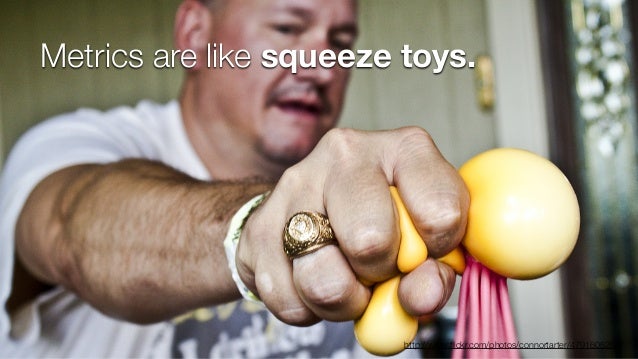In the image, a middle-aged, brawny man is standing slightly off-center, extending his right arm forward. He is dressed in a white t-shirt and sports a gold ring on his ring finger and a white bracelet on his wrist. In his hand, he is squeezing a yellow rubber toy shaped like a person, from which an old, wrinkled pink balloon-like object dangles. The man stands in front of a door with a silver and white frame and a gold handle. The background features a mix of colors including brown, white, tan, yellow, pink, blue, and black. At the top left of the image, there is text that reads, "Metrics are like squeeze toys," suggesting that the image is meant to be a meme or an informational graphic intended for social media.